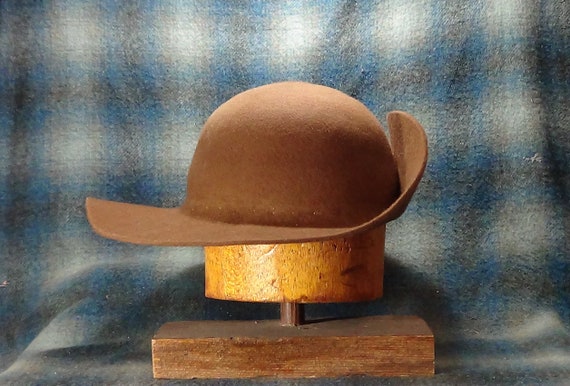This image features a hat resting on a round wooden block, which serves as a display stand. The block is placed on a soft, fabric surface that appears to be blue, white, and black checked, suggesting it might be a blanket or garment. The hat itself sports a unique design where its brim is partially turned up on one side, curving to match the slope of the rest of the hat, while the remaining portion of the brim lies flat. This asymmetrical brim gives the hat a distinct style, combining both functionality for sun protection and an eye-catching, wave-like silhouette.